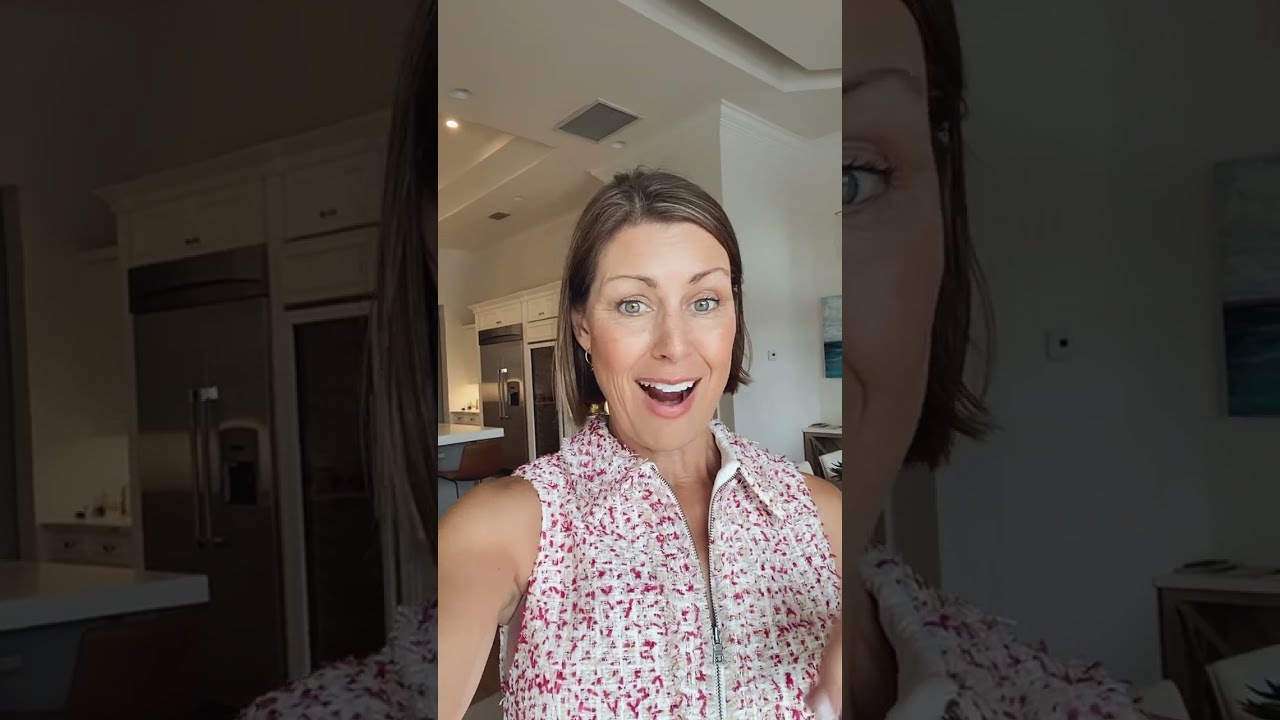The photograph depicts a middle-aged Caucasian woman in her mid-40s with straight brown hair styled in a bob, featuring lighter highlights and parted on the side. She has light blue eyes and is wearing pink lipstick. Her facial expression suggests a mix of surprise and joy, with her mouth agape and eyebrows raised. She is dressed in a white sleeveless top adorned with reddish-pink designs and a central silver zipper.

The background reveals part of her home, specifically her kitchen. Visible elements include a stainless steel refrigerator, white cabinets, a portion of a countertop, and a chair. The overall setting is bright and clear, well-lit by the home's lighting. Notably, the image creatively uses photo editing to enlarge and darken portions of the original image, placing an enhanced view of the refrigerator on the left and a close-up of the right side of her face on the right as borders. There are no other people, text, or numbers in the image. The photograph captures a moment of evident happiness and cleanliness in her home.